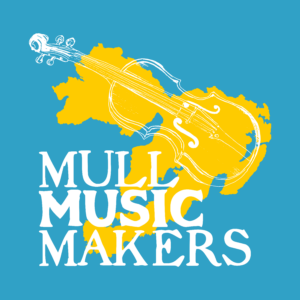The image features a graphic design with a solid light blue, almost turquoise background. At its center is a yellow shape resembling an island or country, over which a white outline of a violin is superimposed. The shape of the violin appears to align with the contours of the yellow figure. Centered towards the bottom of this image, the text "Mull Music Makers" is prominently displayed in bold white letters. The first letter of each word aligns vertically, with "Music" standing out more boldly compared to "Mull" and "Makers". The overall composition, with the violin outline and bold text, suggests an advertisement or logo.